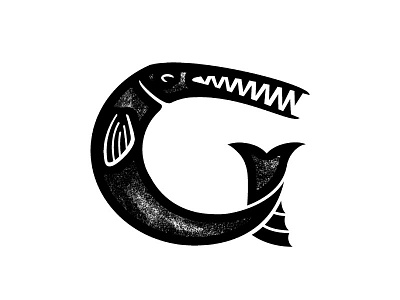The image showcases a detailed, black and white sketch of a sea creature, possibly resembling an eel or barracuda, set against a solid white background. The creature is depicted in a side profile, with its body curving gracefully into the shape of a capital C or G. Its long, beak-like mouth is lined with jagged, razor-sharp teeth, slightly open to reveal the menacing interior. The creature's solitary eye and fins are meticulously outlined in white, with additional white streaks accentuating the ridges and texture of its body, particularly around the neck and tail sections. The sketch appears rich and dark with subtle smudging, adding to the vintage, hand-drawn aesthetic of the design.